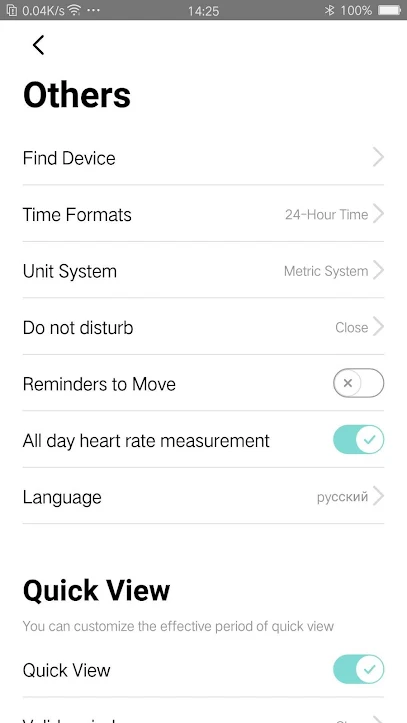This image is a screenshot of a device settings menu. In the upper left corner, there is a heading labeled "Others." Below this heading, various options are listed in a vertical column. The options are as follows from top to bottom:

1. **Find Device**
2. **Time Formats**
   - **24-hour time**
3. **Unit System**
   - **Metric System**
4. **Do Not Disturb**
   - Status: On (closed)
5. **Reminders to Move**
   - Status: Off
6. **All Day Heart Rate Measurement**
   - Status: On

A section is also present where the language setting displays non-English characters resembling "P Y C C K," two backwards "N"s, and a character with a squiggly line above it. Below this language section, there is another section with a bold title labeled "Quick View." This section provides a description stating, "You can customize the effective period of Quick View." Beneath the description, the setting is listed once more as "Quick View."

A gray arrow points to the right on all these settings, indicating that more options can be accessed. The screenshot shows the device battery at 100% and the current time as 14:25 (2:25 PM).